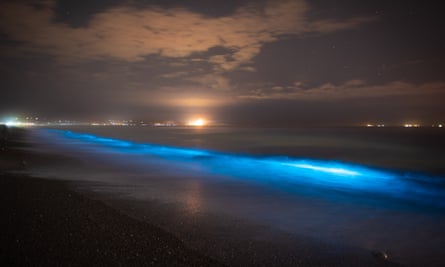The image captures a mesmerizing night scene at the beach, where the remnants of dusk cast a soft glow on flat, thin clouds with a light pink hue. The horizon features distant city lights mingling with the barely visible sun as it sets. Bright blue bioluminescent waves, strikingly illuminated, lap against the shore, leaving the wet sand glistening and reflective. The foreground remains shrouded in darkness, enhancing the ethereal quality of the bioluminescent tide. Clouds are depicted in two distinct groupings, with the larger one closer and the thinner one fading into the distant horizon. Pebbles are scattered across the beach, adding texture to the serene and captivating coastal tableau.